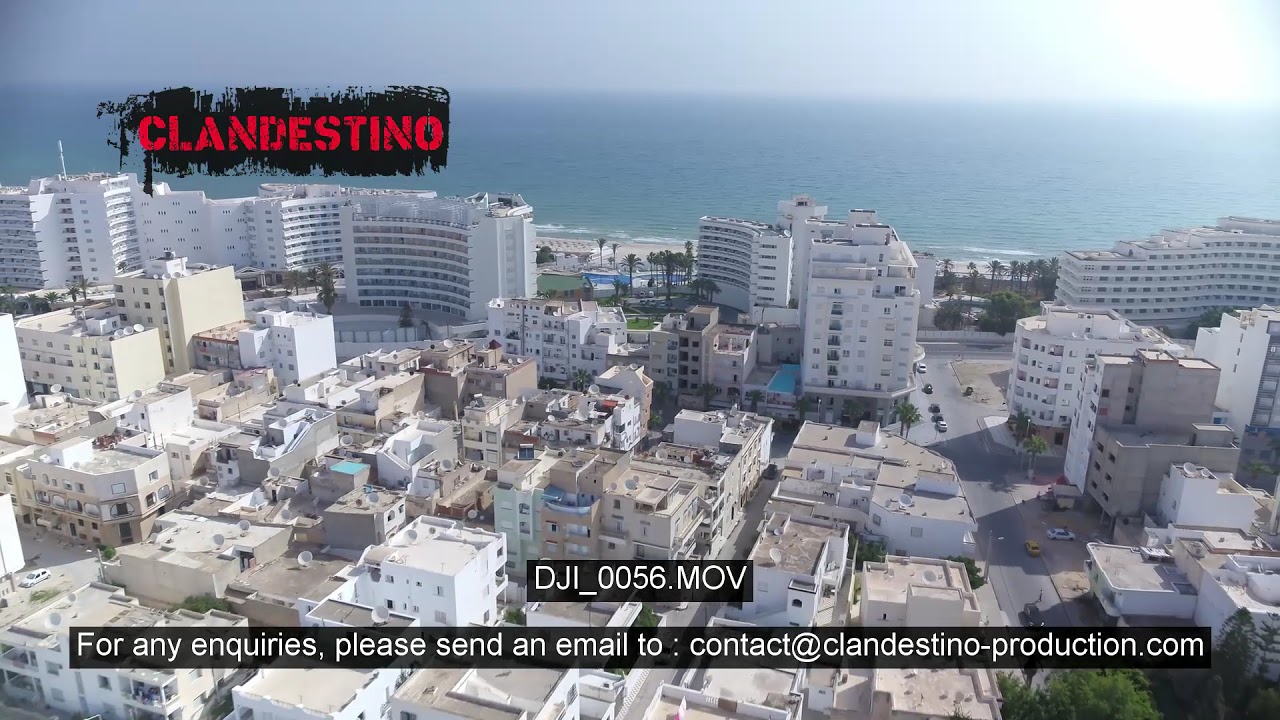This detailed, landscape-oriented, aerial photograph captures a bustling cityscape bathed in daylight. The central focus reveals a densely packed urban environment marked by a variety of multi-story buildings, potentially a mix of residential and commercial properties. The structures predominantly feature light colors such as white, beige, and tan. The foreground buildings are aligned closely together, with a prominent roadway visible on the right-hand side extending towards a vast, light blue ocean occupying the top third of the image. 

Adjacent to the ocean, we see a large, curved building that might be a hotel or condominium complex, adding a notable landmark to the scenery. The photograph, likely taken by a drone or from atop a high building, offers a downward perspective that accentuates the extensive urban sprawl. 

In the top left corner, an inked-out rectangular area bears the word "CLANDESTINO" in a red, stamped font. At the bottom of the image, "DJI-0056.MOV" is inscribed in white text, accompanied by a contact email for inquiries: contact@clandestinoproduction.com. The composition captures both the city and the seascape, illustrating a harmonious blend of urban and natural elements under a clear, sunny sky, representative of photographic realism.